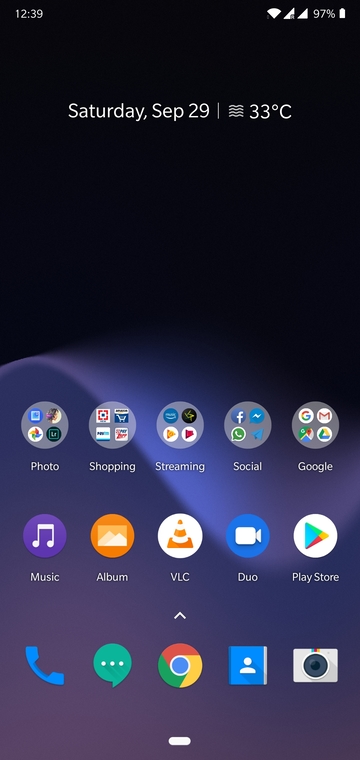A detailed screen capture from someone's cell phone front screen. At the top, the status bar displays the time as 12:39, along with a Wi-Fi signal indicator and a cellular signal indicator. Beside these, it shows the battery level at 97% with a small battery icon. Below the status bar, the date reads "Saturday, September 29" and the temperature is indicated as 33 degrees Celsius. 

At the bottom of the screen, a row of app folders is visible, labeled as "Photoshopping," "Streaming," "Social," and "Google." Below these folders, several individual app icons are displayed, including Music, Album, VLC, Duo, Play Store, Phone, Chat, Google Chrome, Contacts, and Photos.

The background of the cell phone features a dark and mysterious design, with a black base color complemented by a wavy blue and purple pattern that adds a misty and ethereal effect. This screen capture provides a comprehensive view of the various apps organized on the person's home screen, set against a strikingly enigmatic background.